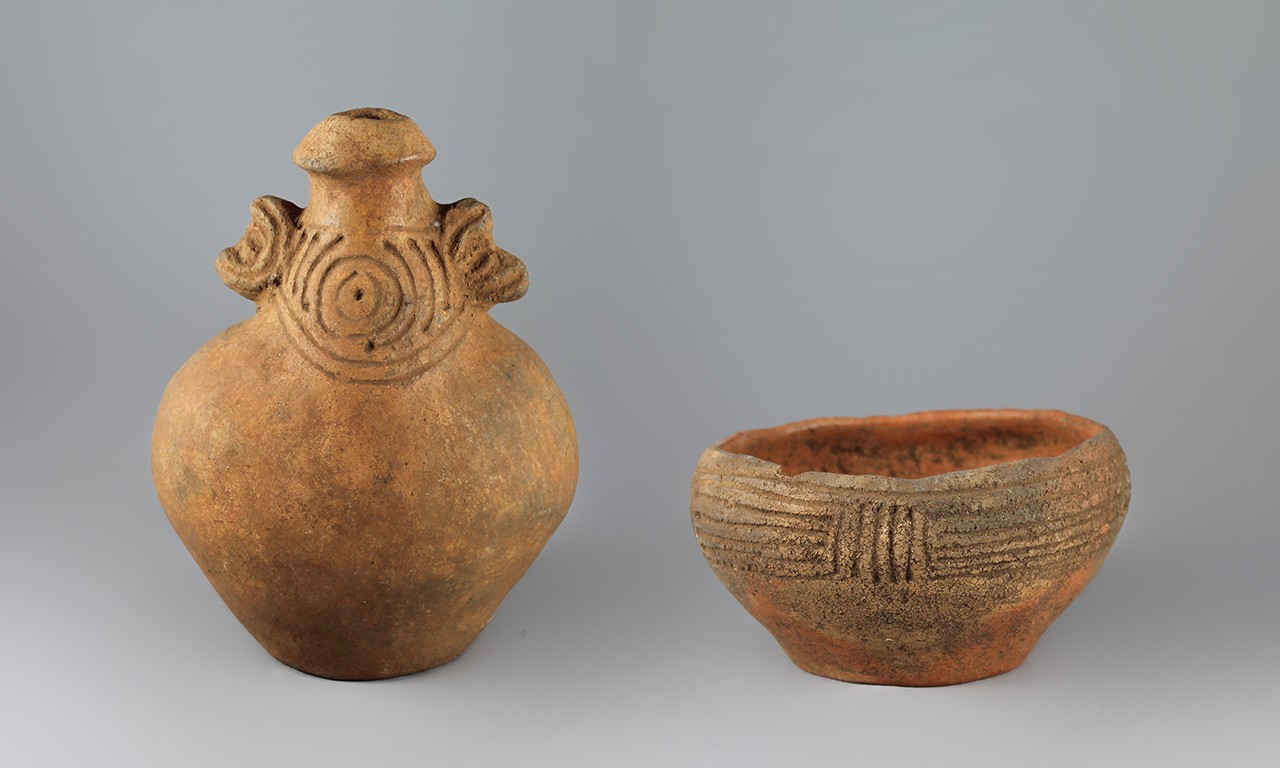The photograph, taken in a professionally lit studio and set against a blank, white background, features two ancient-looking pottery pieces made of clay or terracotta. On the left is a jug-shaped vase with a bulbous base that narrows into a round neck with a small opening, indicative of its possible use for holding liquids like wine or water. This vase has etchings around its neck and includes small handles on its sides, adding to its historical charm. On the right is a deep ceramic bowl with a noticeable rough texture, suggesting it may not have been fully fired in a kiln. The bowl has a smaller base that widens into a broad, flat opening, with line engravings adorning its upper half. It also has a slight chip on the front left side, adding to its weathered appearance. Both pieces share a clay color and an aged, worn look that evokes the sense of artifacts discovered at an archaeological site.